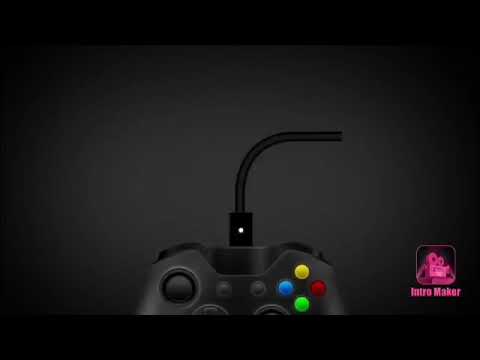The image is a detailed 3D render of a Microsoft Xbox controller viewed from above, positioned towards the center of a rectangular frame. The Xbox controller is primarily black with distinctive color-coded buttons: yellow at the top, blue on the left, green on the bottom, and red on the right. In the center of the controller, there are two equally sized buttons, with a significantly larger black button situated to the left. The controller features shoulder triggers and hints of the top analog stick, though the D-pad and lower analog stick are cropped out of the image. An antenna-like black USB cable is plugged into the controller, curving toward the right, with a small white LED light appearing at the end of the cable.

The background of the image transitions from gray to black, with black borders on the top and bottom edges. To the right of the controller, there’s a pink logo labeled "Intro Maker," featuring a small symbol that resembles a robot. This detailed depiction emphasizes the controller’s design and the USB charging feature, highlighted by the glowing LED indicator.